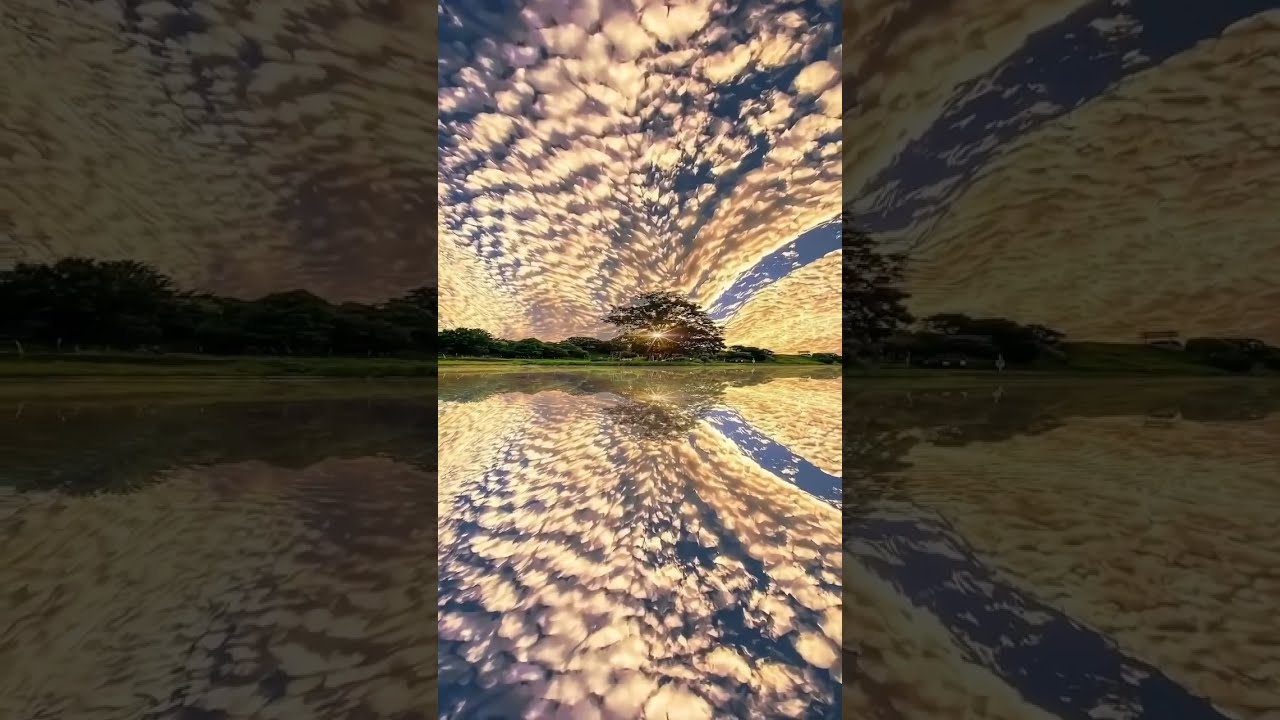The image showcases a digitally enhanced landscape captured in three vertical sections; the left and right bars are shrouded in dark hues, while the central bar is vividly bright, almost as if a light is shining directly onto it. The central image, nearly 2 inches wide within the 8x5 inch photograph, features a breathtaking scene of a large tree on a background landmass. The low-hanging Sun casts a golden glow across the sky, with its rays piercing through the branches of the tree. Feathered, fluffy clouds stretch across the blue sky, perfectly mirrored on the tranquil surface of a lake below, creating a striking symmetry. The landscape, including the blue sky, yellow clouds, and lush greenery, is flawlessly reflected in the water, enhancing the serene and idyllic atmosphere of the scene.